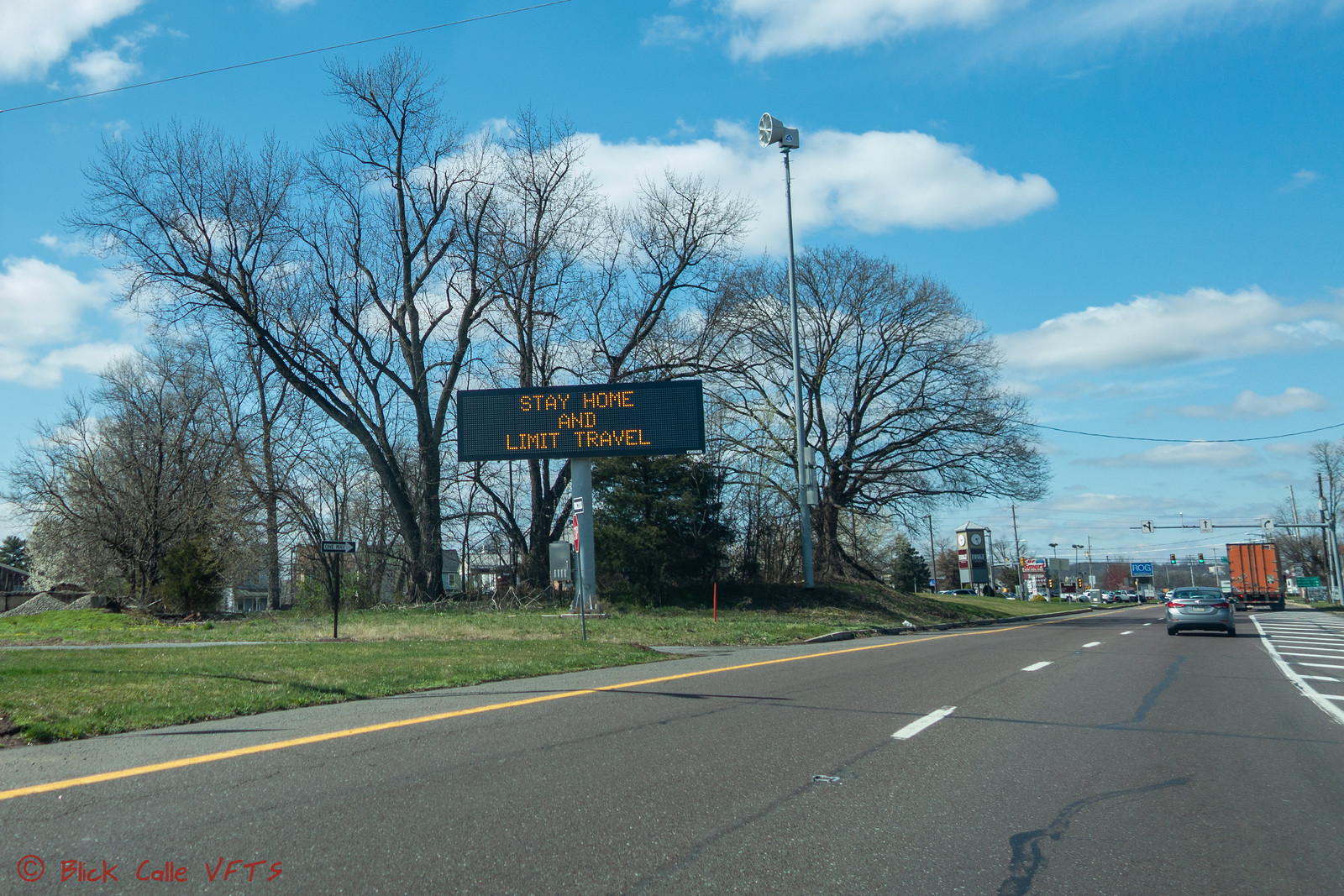The image captures a two-lane street, likely one-way, with sparse grass and some large, leafless trees on a sunny day with clear blue skies and fluffy white clouds. In the foreground, there are vehicles, including a semi-truck and a car. To the left of the road, an electric marquee sign with black and yellow lights reads "Stay Home and Limit Travel," likely from the COVID era. The street features minimal traffic and leads into a small town or city dotted with storefronts and buildings. A sidewalk, a grassy area, and numerous signs and power lines are visible, adding to the urban landscape.